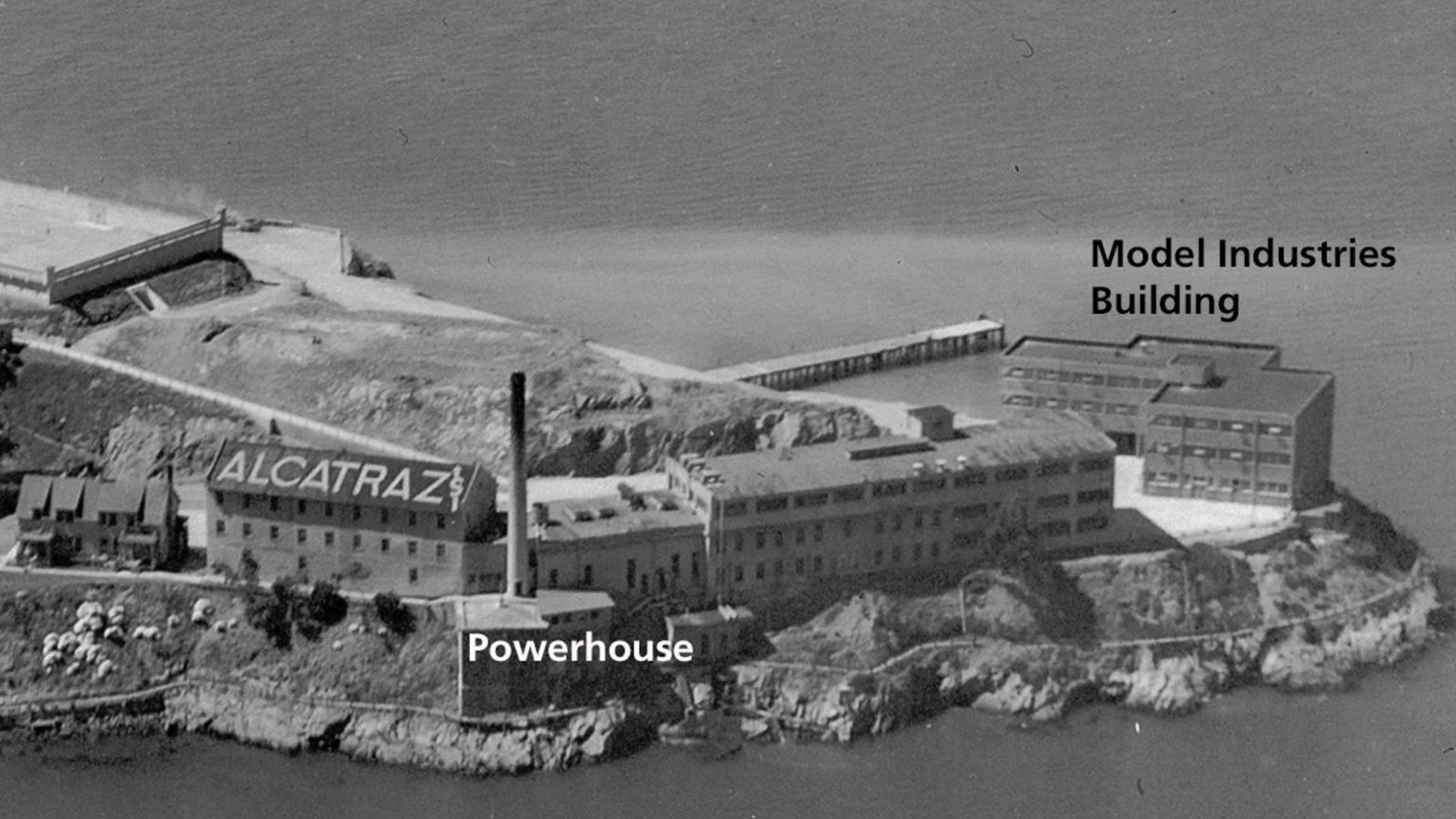This monochromatic photograph depicts a realistic model of Alcatraz Island, with clear views of significant buildings. The island, surrounded by gray water and rocky cliffs, features prominently in the center of the image. A long, three-story main building stretches from just left of center toward the right, proudly displaying the word "Alcatraz" on its roof. To the right of this structure, another building is labeled "Model Industries Building," indicative of its purpose during the penitentiary's operation. In front of "Alcatraz," the term "Powerhouse" is visible with a chimney rising upward, suggesting utilities infrastructure. A dock extends from the center out into the water, underlining the island's isolation. Scattered trees and grassy areas add texture to the left side of the image, creating a stark contrast to the somber tones of the island's imposing architecture.